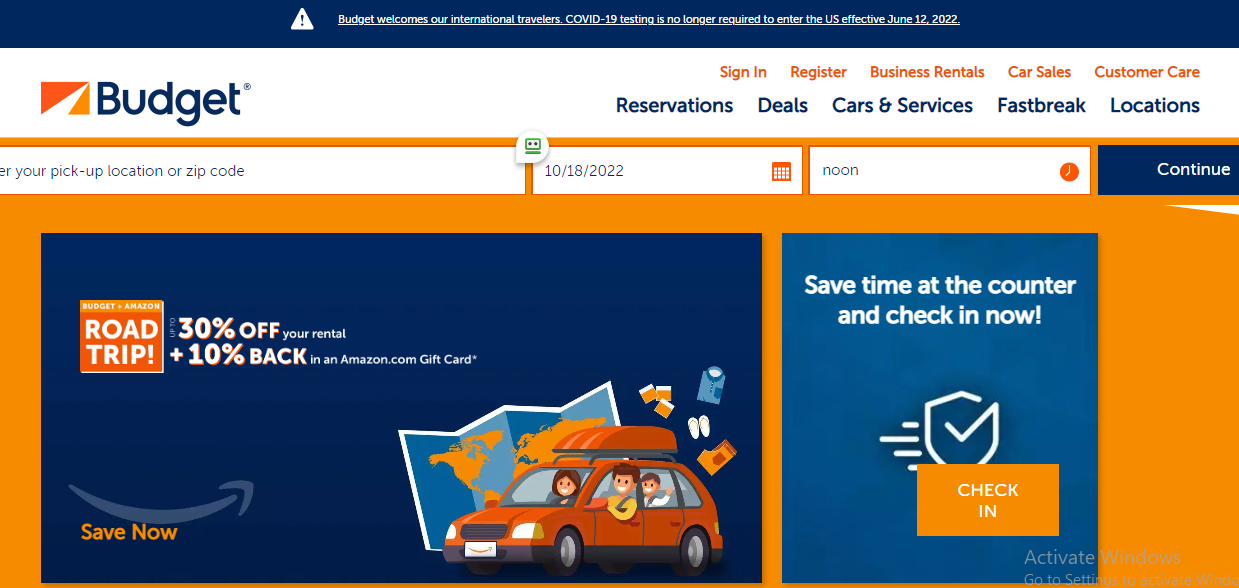The desktop homepage of Budget Car Rentals features a prominent logo at the top left, consisting of two converging orange triangles that form the visual impression of a road leading into the distance. A welcoming message for international travelers is displayed at the top, noting that COVID-19 testing is no longer required to enter the U.S. effective June 12, 2022. Below this announcement are fields to input your pickup location or zip code, select dates from a calendar, and choose a time for your rental. A graphical illustration below these fields depicts a cartoon family in a car with a camper shell on top, promoting a "Road Trip" discount: 30% off rentals plus a 10% cashback in an Amazon.com gift card. The overall color scheme predominantly features orange and white.